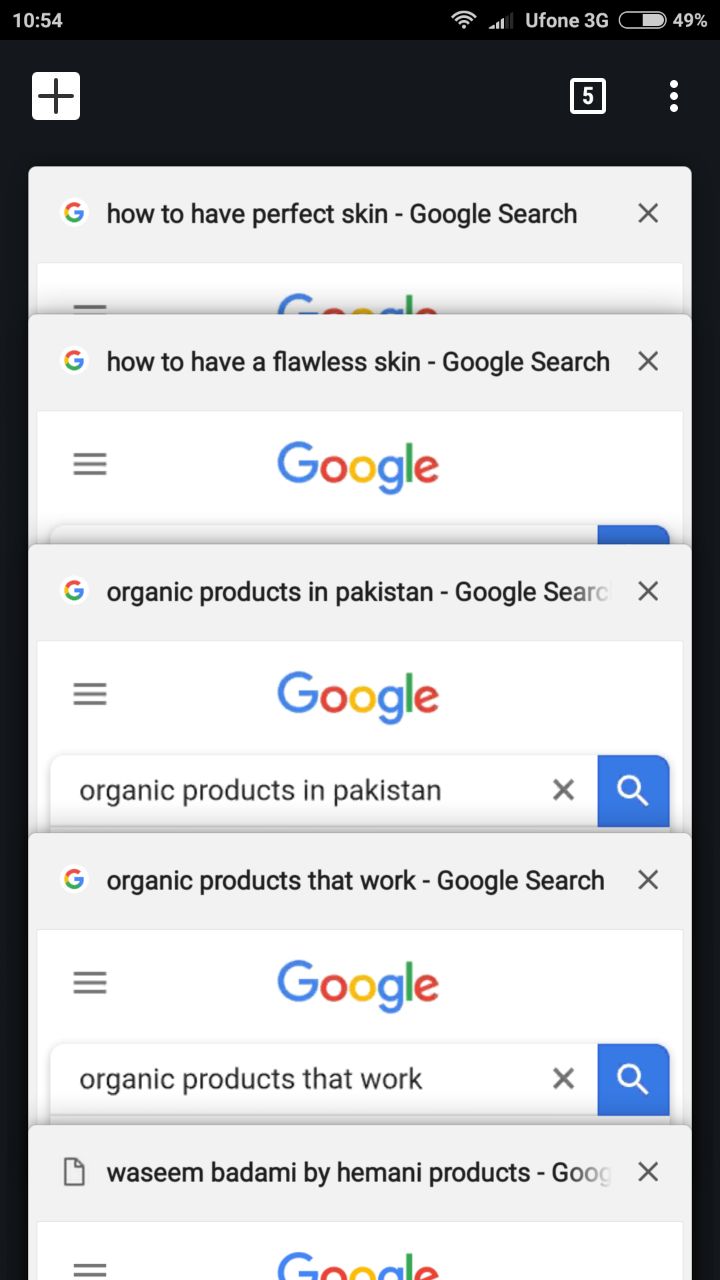In this image, we observe a cell phone screen displaying multiple open windows. The phone's status bar at the top shows the current time, Wi-Fi signal, and battery meter, identifying it as a mobile device. Below the status bar, on a black background, there is a white tab indicating the number '5' within a box, suggesting that five windows are currently open. All these windows are Google search results, as evidenced by the typical white Google search box with the Google logo at the top of each window. 

The first search result at the top reads, "How to have perfect skin," followed by another query, "How to have flawless skin." The subsequent searches include "Organic products in Pakistan," "Organic products that work," and "Wasim Badami by Himani Products." These searches indicate a focus on skincare, highlighting an interest in achieving perfect skin and exploring effective organic skincare products, including specific items by Wasim Badami.